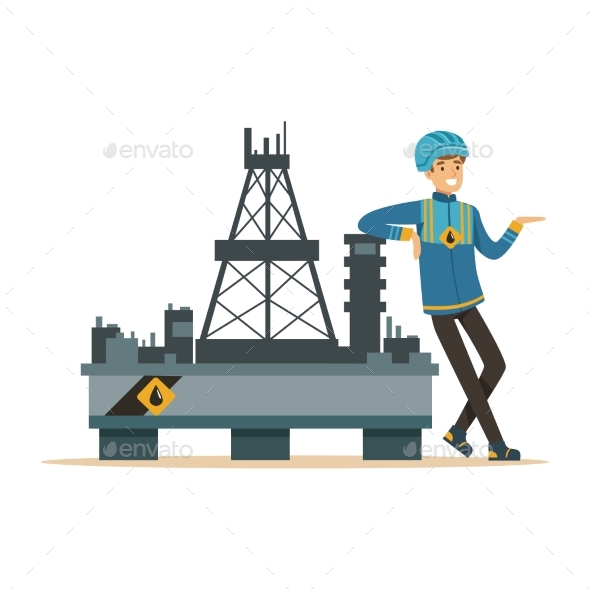The digitally-created graphic image showcases a vector illustration of a cartoon man positioned on the right-hand side. The man, sporting a blue helmet and a smile, is dressed in a blue and yellow jacket featuring a black oil drop symbol within a diamond on the chest. He also wears black trousers and grey and yellow shoes. The man is casually leaning against a small model oil rig situated in the center of the image. This oil rig, depicted with intricate details, stands on a light brown oval base and has three legs supporting a structure with rectangular towers, a triangular spire, and various blocks in different shades of gray. A diagonal black line runs along the face of the oil rig, which also includes a diamond with a black oil symbol inside it.

The background is predominantly solid white, overlaid with a watermark comprising diagonal broken light gray lines that form a diamond grid pattern. In addition, the background features multiple instances of the word "Envato" in a greyed-out font, appearing in the top left, top right, bottom left, and bottom right corners of the image. The watermark text and a leaf-like symbol to the left of the word "Envato" enhance the graphic’s distinctive stock image appearance.